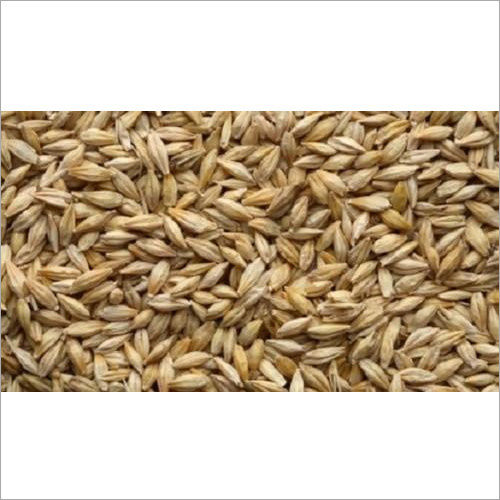The image is set within a rectangular frame bordered by a thin, dark grey line. The background is a pristine white, and the image also features white bands at the top and bottom quarters of the frame. Dominating the center of the image is a dense cluster of oval-shaped seeds, possibly oats or grains, characterized by a range of beige, light yellow, and brown shades. The individual seeds, which have pointy ends, are oriented in various directions, creating a visually textured and shadowed composition. The absence of contextual elements and the uniformity of the seeds emphasize their collective form, making them the focal point against the minimalistic background.